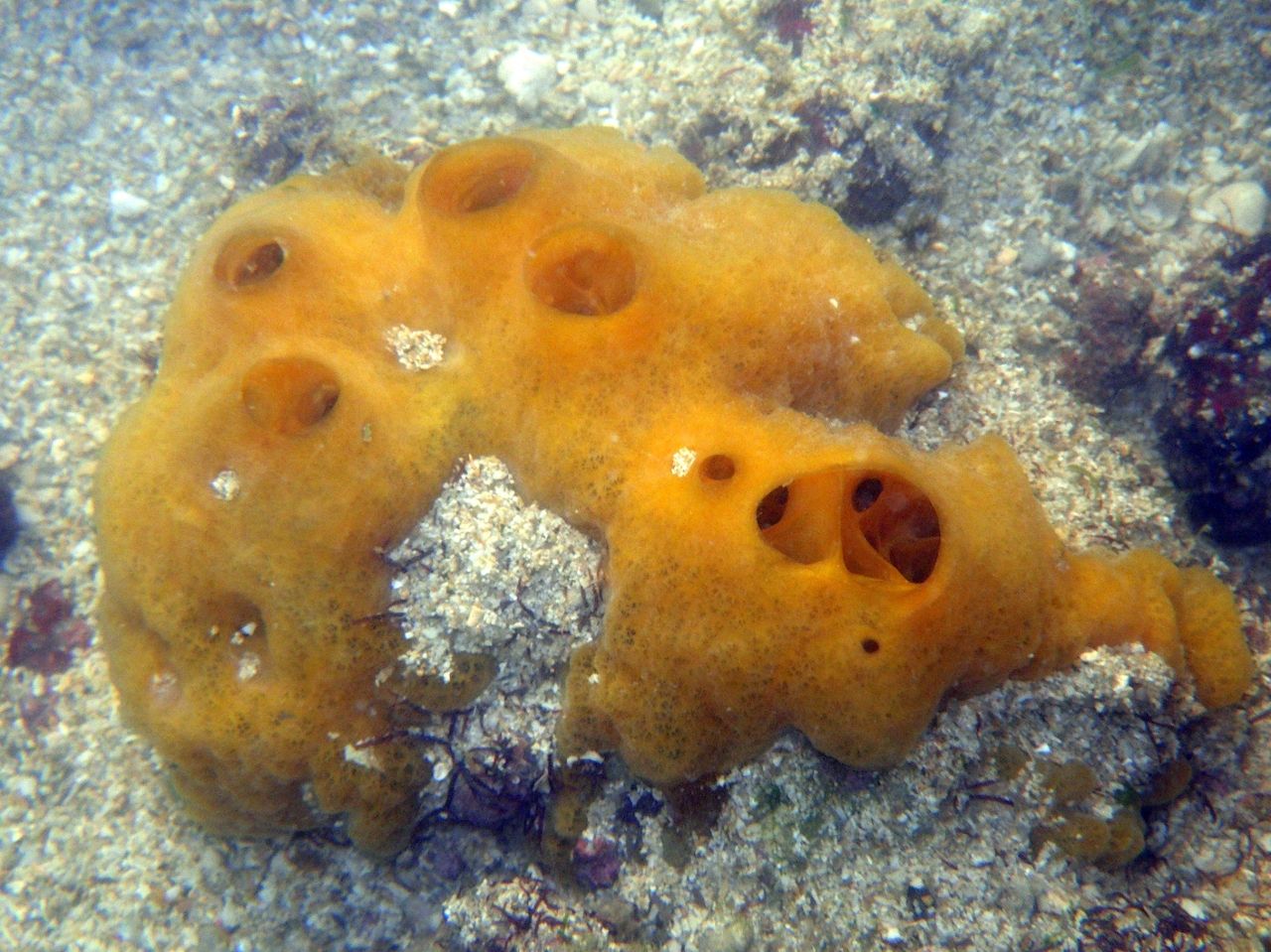This photograph captures an underwater scene featuring a prominent, yellow, porous structure—likely a coral or sponge—situated at the center of the image. The sponge-like entity is characterized by numerous small holes and several larger chambers, giving it a distinctly pitted appearance. Its yellow hue stands out vividly against the surrounding environment, which predominantly consists of a sandy seabed sprinkled with various sediments, including small rocks and pebbles. A fine layer of this sediment appears to have settled atop the sponge in some areas. The photograph reveals a clear, transparent body of water, suggesting it was taken in shallow depths, possibly under daylight, as indicated by the light illuminating the rocks and sand. The overall composition lacks any textual information, and colors in the image range across the spectrum, including black, white, shades of gray, tan, maroon, orange, and yellow. The scene is a static snapshot of the ocean floor, emphasizing the natural and undisturbed underwater habitat.